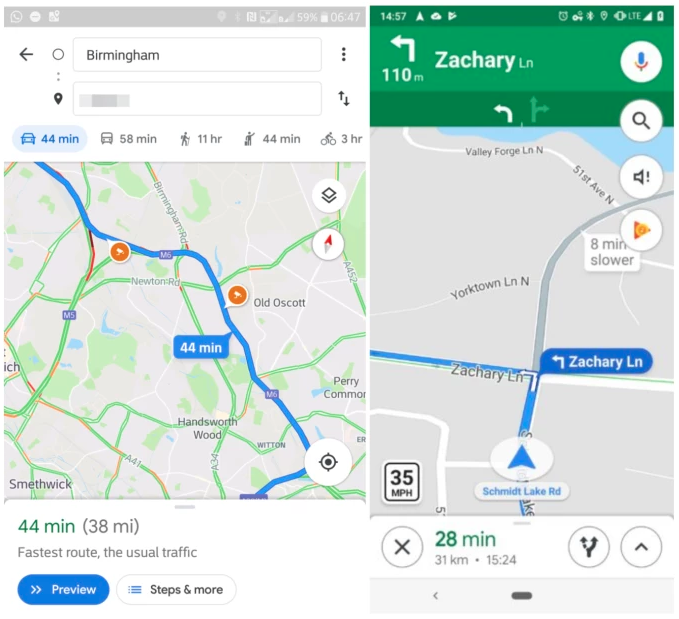The image consists of two detailed screenshots from a smartphone, each depicting navigation information.

On the left screenshot, at the top of the screen, there is a gray border with white icons indicating it is 6:47 AM and the battery is at 59%. The interface appears to be from Google Maps or a similar application. The top search bar shows "Birmingham" as the input, while the destination field is either empty or obscured by a gray bar. The app is displaying transportation options: by car (44 minutes in blue, selected), bus (58 minutes, gray), walking (11 hours, gray), hitchhiking (44 minutes, gray, represented by an icon of a person with a thumb out), and bicycle (3 hours, gray). Below these options, a map is shown with notable towns such as Old Oscot, Handsworth Wood, Perry Common, and Smithwick (bottom southwest corner). A thick, wavy blue line runs from the top left to the lower right, indicating a main road. Smaller roads are highlighted in green, and red pins likely mark the start and destination points. Below the map, there’s a note stating "44 minutes, 38 miles, fastest route, usual traffic" along with buttons labeled "Preview" and "Steps and more."

The right screenshot has a green header displaying the time 2:57 PM (14:57) and usual status icons for battery and signal strength. The screen shows a turn-by-turn navigation interface, indicating the user needs to turn left onto Zachary Lane in 110 meters. The current location is on Schmidt Lake Road, visualized with an arrow showing the direction of travel. The speed limit is 35 miles per hour, suggesting a residential area. At the bottom, it mentions "28 minutes, 31 kilometers, 15:24" with an "X" button for canceling and other icons for modifying the directions.

This comprehensive navigation scenario likely takes place in the UK, given the town names and the presence of a main road cutting through multiple locales.